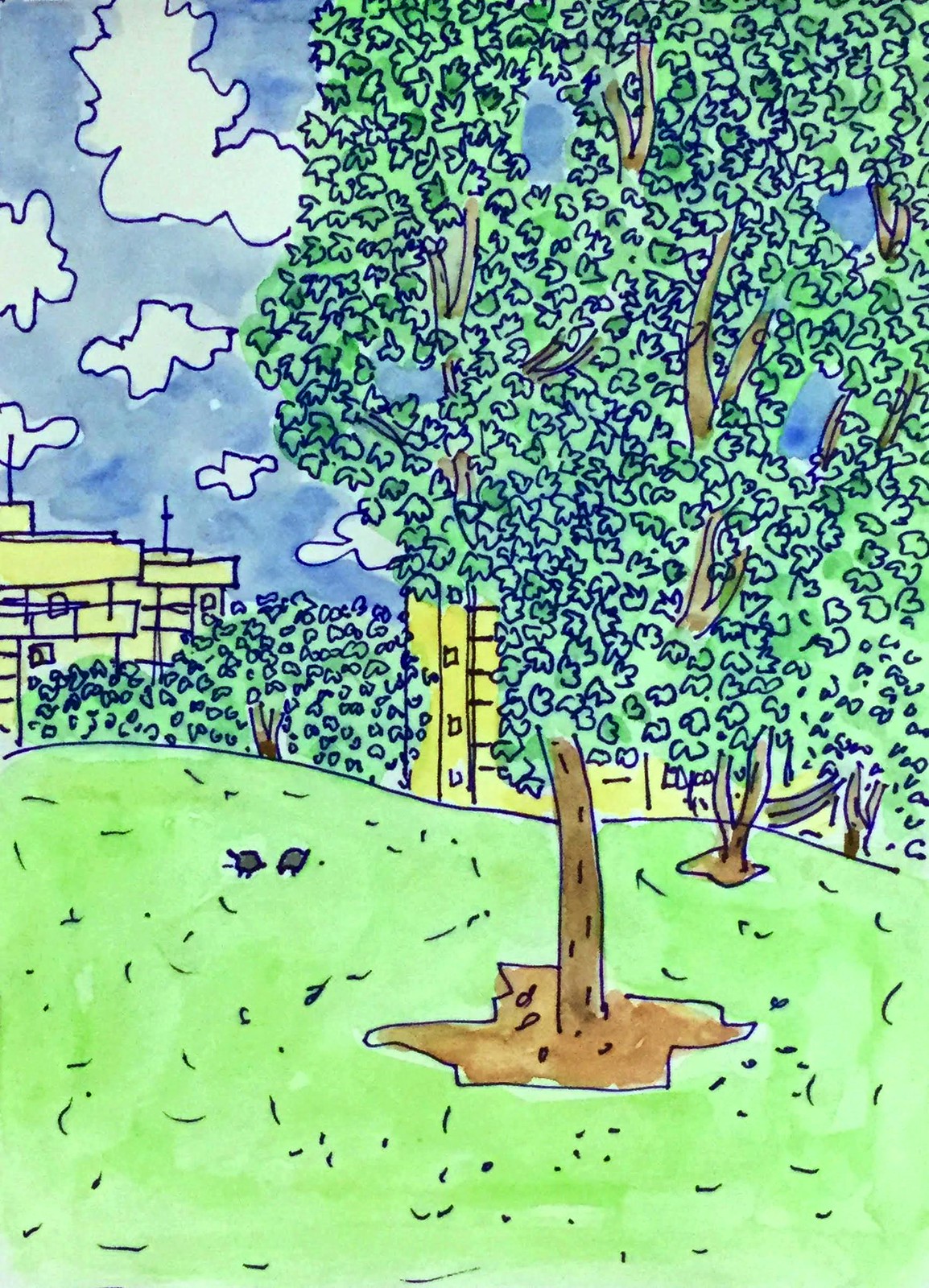This watercolor painting captures a serene landscape featuring a prominent tree in the foreground. Adjacent to this main tree is another tree positioned on a small hill, creating a sense of depth. In the background, at least two more trees are visible over the edge of the hill, adding layers to the composition. Beyond the trees, multi-story buildings rise, some topped with what appear to be weather poles or antennas. The sky is a clear, light blue, dotted with soft white clouds. The trunks of the trees are rooted in patches of bare dirt, which transition into lush green grass. Two birds, rendered in light gray with black outlines, soar gracefully in the sky, completing the tranquil scene.